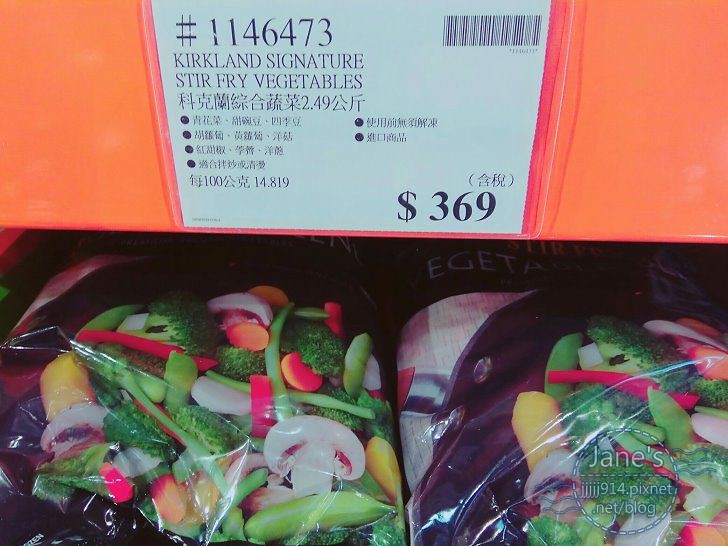This photograph captures two large bags of Kirkland Signature Stir Fry Vegetables displayed in a grocery store. The top of the image prominently features the product name "1146473 Kirkland Signature Stir Fry Vegetables" alongside several sentences written in an Asian language. Each bag contains an assortment of vegetables, including mushrooms, broccoli, carrots, string beans, red cabbage, yellow squash, and red bell pepper, suggesting a substantial mix suitable for stir-fry dishes. The price tag, clearly visible in the bottom right corner, shows $3.69. The frozen vegetables are set against an orange background flanking a white sign with the price. No people are present in the photograph, keeping the focus solely on the products. A small barcode is also visible, emphasizing the retail setting.